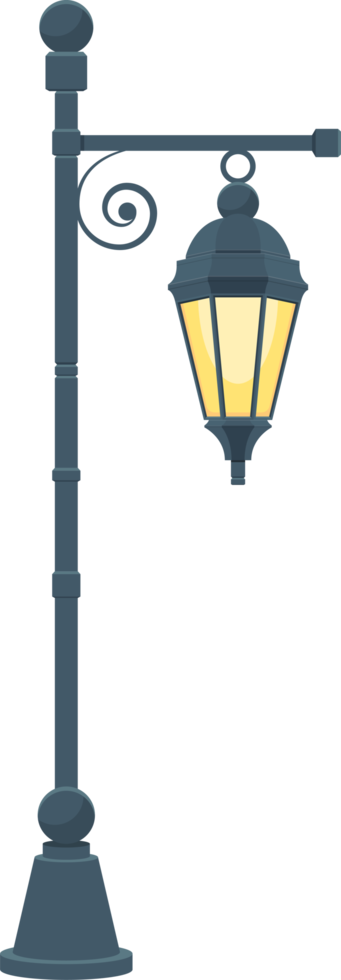The image depicts a clip art illustration of a vintage street lamp centered against a pure white background. The street lamp features a steely, dark gray base— a mix of blue and gray tones. Rising about four feet tall, the lamp stand has an ornamental circle near its top, from which a horizontal handle stretches out, suspending a lantern. The lantern itself has three glass panes through which a yellow bulb emits a muted light that does not extend beyond the lamp. The glass panes are accented with subtle blue lines, adding to the lamp's detailed aesthetic. Despite its simplicity and lack of vibrant colors, the detailed design evokes the charm of an old-time street lamp.